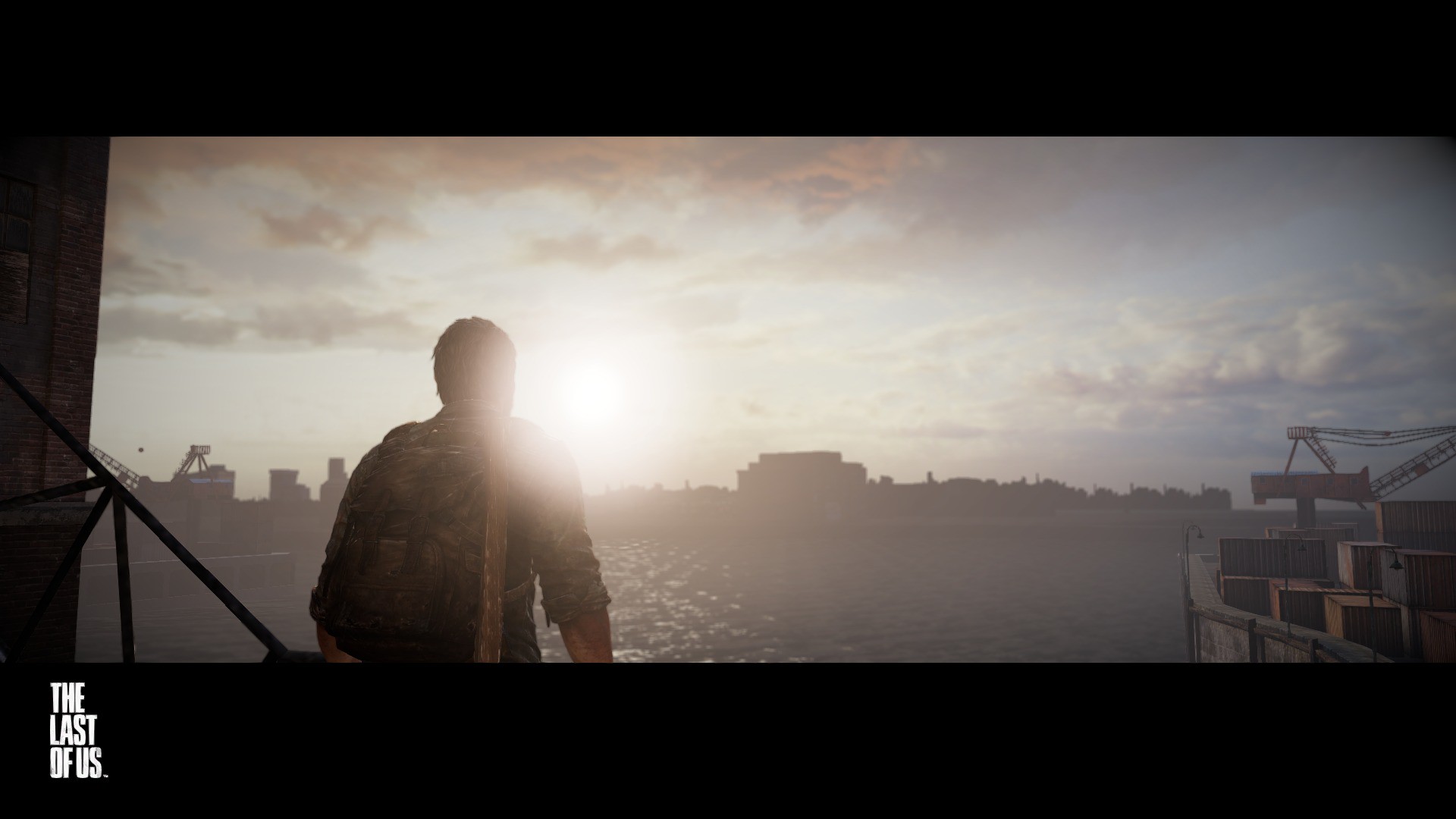The image is a detailed screenshot from the video game The Last of Us, depicted in a landscape mode with a wide, dark border. In the bottom left-hand corner of the border, the title "The Last of Us" is displayed in white type. The focal point of the screenshot is the back view of Joel, a main character from the game, standing in the foreground. He is dressed in a camouflage shirt with sleeves rolled up to his elbows, carrying a backpack and an axe. Joel appears to be gazing at a picturesque sunset over a body of water, with clouds scattered across the sky. To the left of the scene, there's a wooden structure with some boxes, possibly the side of a boat. In the distance, beyond the water, a cityscape with buildings is visible, and to the right, a freighter loaded with shipping containers can be seen. The overall composition beautifully captures a moment of calm and introspection in the game's post-apocalyptic setting.